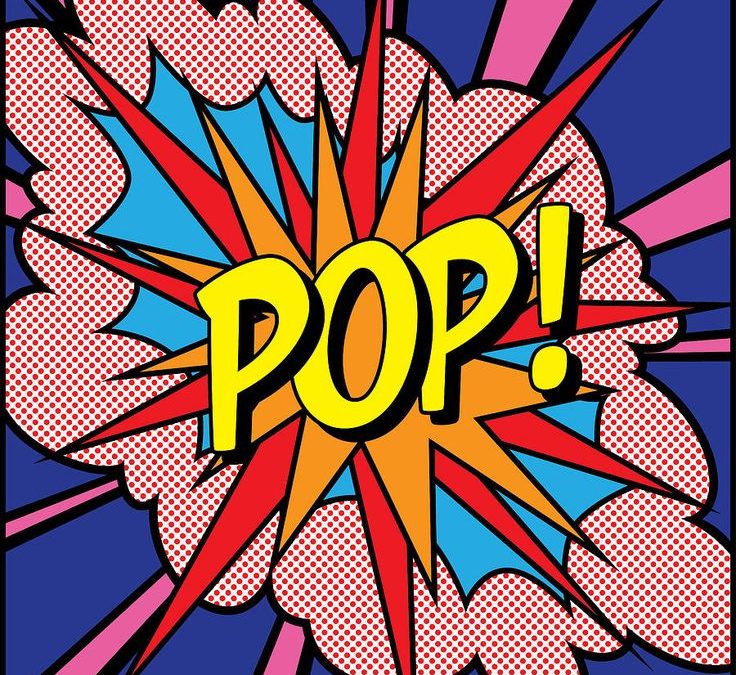This detailed digital image is reminiscent of classic comic book style, showcasing a sound effect commonly seen when characters punch or kick, similar to the old Batman TV show. The central focus of the image is the bold, bright yellow word "POP!" with an exclamation point, rendered in comic book-style lettering with black shadows, making it appear three-dimensional and as if it's popping out towards you. Behind the word "POP!" is a vibrant explosion with multiple spiky layers: the innermost part is bright blue encircled by a white cloud speckled with red polka dots, followed by an intense mix of reds and oranges. The background is dramatic with purple and pink radial stripes emanating outward, giving the impression of a dynamic, bursting effect. The extreme background features bold purple rays outlined in black against a navy blue fill, enhancing the explosive impact of the central imagery. This intricate and vivid representation effectively captures the high-energy and visually striking elements characteristic of comic book onomatopoeia.